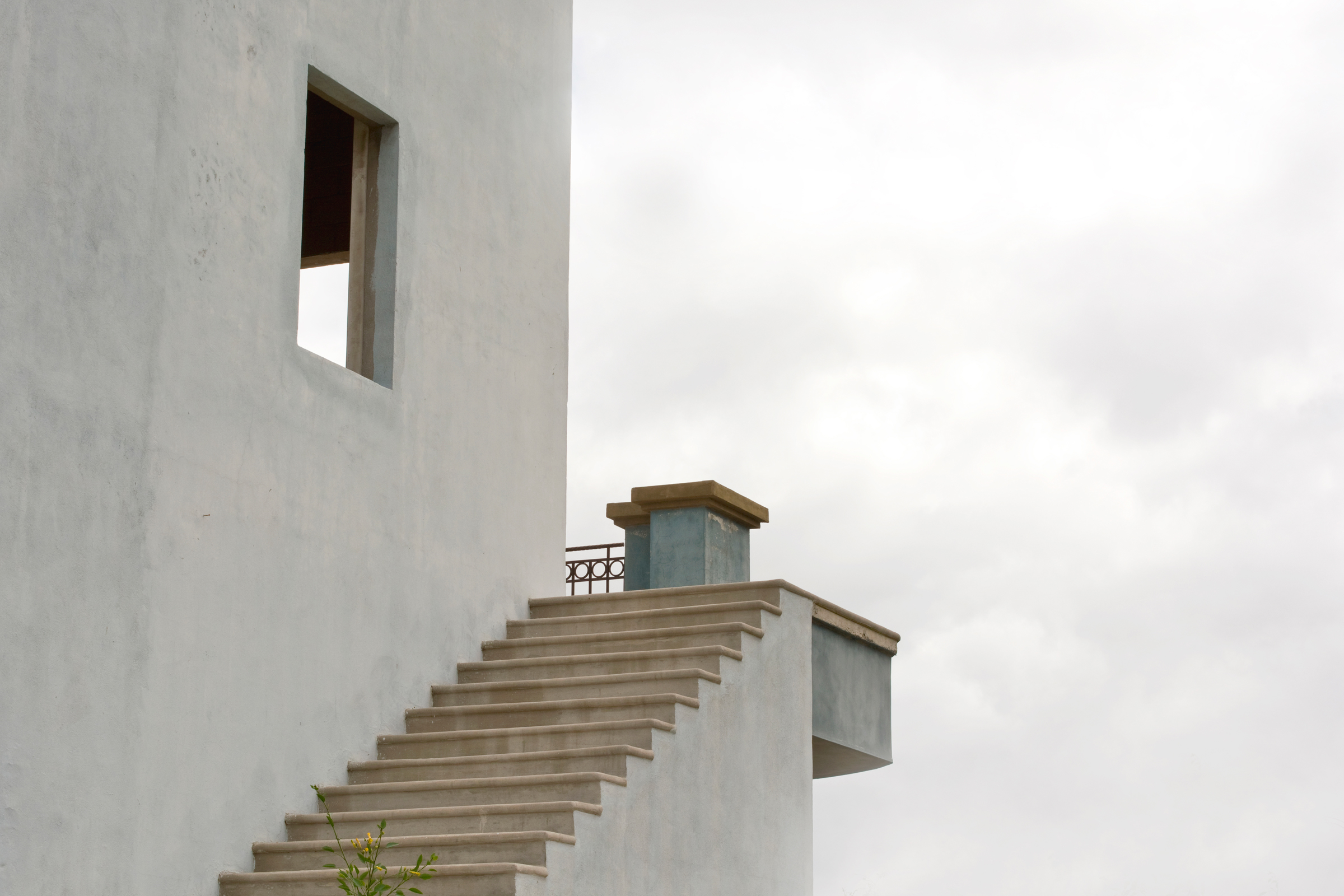The image features a white, possibly illustrated or video game scene depicting an unfinished, masonry building with a smooth, cement exterior that evokes a Middle Eastern vibe reminiscent of a few centuries ago. The right side is a light tan, empty background enhancing the focus on the left where a wide, cement staircase without a railing ascends approximately 15 steps. The steps are quite wide but appear shallow and lead up to a small balcony or patio area featuring bronze and gray-green hues. Behind the balcony, a hint of a wrought iron railing is visible. The building itself exhibits tan plaster with brick accents, particularly around the staircase. There are two unglazed, unframed windows positioned catty-corner to each other, providing a glimpse into the unfinished interior, revealing wooden beams or framing. A small plant grows at the base of the stairs. The setting is under a hazy, gloomy sky, adding to the overall atmosphere.